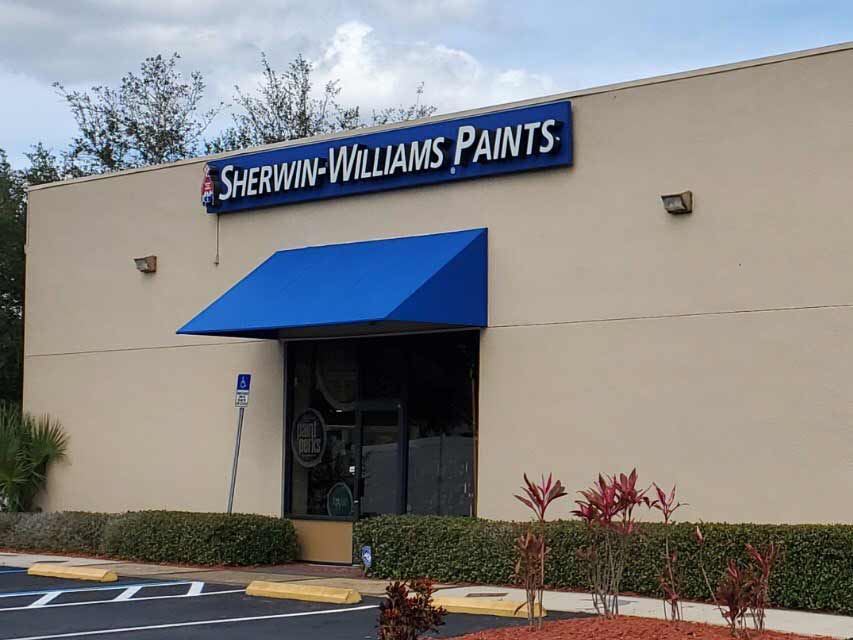The photograph depicts the storefront of a Sherwin-Williams Paint Store, positioned at a slight diagonal angle with the right side sloping slightly lower than the left. The building features a tan cement facade, crowned by a long, dark blue horizontal sign that boldly displays "Sherwin-Williams Paints" in large, white, uppercase letters. On the far left edge of the sign, an upturned red paint can is depicted, from which red paint appears to be pouring out.

Beneath the prominent sign is a blue canvas awning, shading a set of double smoky gray doors. To the left of the doors stands a silver pole with a white and blue handicapped parking sign attached. Above the awning, positioned both on the left and right sides, are matching spotlights that illuminate the store's entrance.

A series of neatly trimmed hedges lines the edge of the sidewalk that runs horizontally in front of the store. At the bottom right corner of the scene, there is a red mulch mound adorned with reddish-colored flowers. Adjacent to the mound, an expanse of dark asphalt marked with white lines delineates parking spaces, each outlined by a yellow cement parking barrier just before the sidewalk.